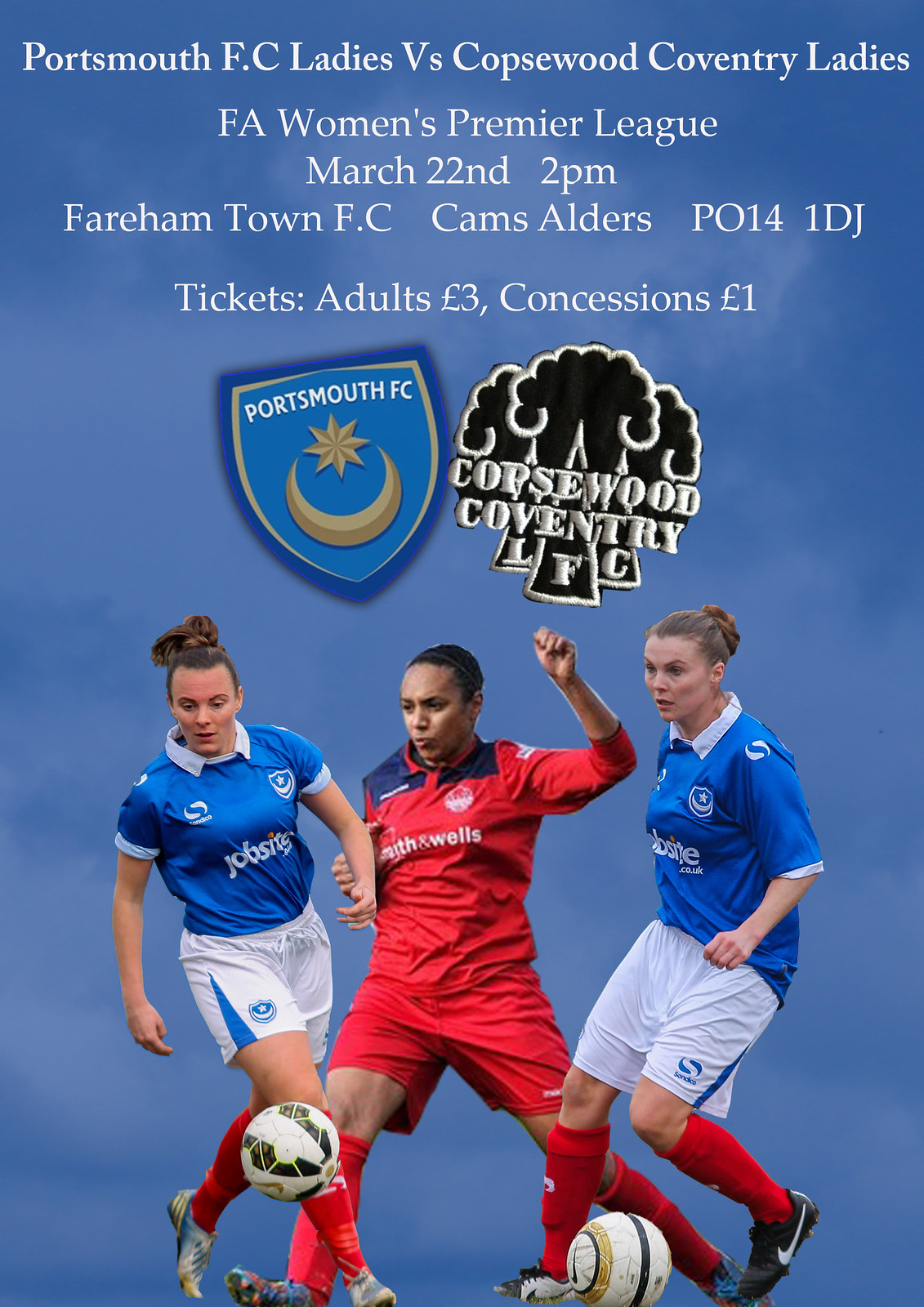The image is a poster advertising a soccer match, set against a textured blue background. At the top, in white text, it reads: "Portsmouth F.C. Ladies vs. Copeswood Coventry Ladies, F.A. Women's Premier League, March 22nd, 2 p.m.," followed by "Fairham Town F.C., Cams Elders, PO14 1DJ." The next line details ticket prices: "Tickets: Adults £3, Concessions £1." The poster features two logos, one representing Portsmouth F.C. with a yellow crescent moon, and another for Copeswood Coventry F.C. with distinctive green, white, and black elements. At the bottom, three female soccer players are shown in action: two in white shorts and blue tops, flanking a player in a red outfit. Two soccer balls are visible in the scene. The overall layout has the text predominantly at the top and the dynamic image of the players at the bottom.